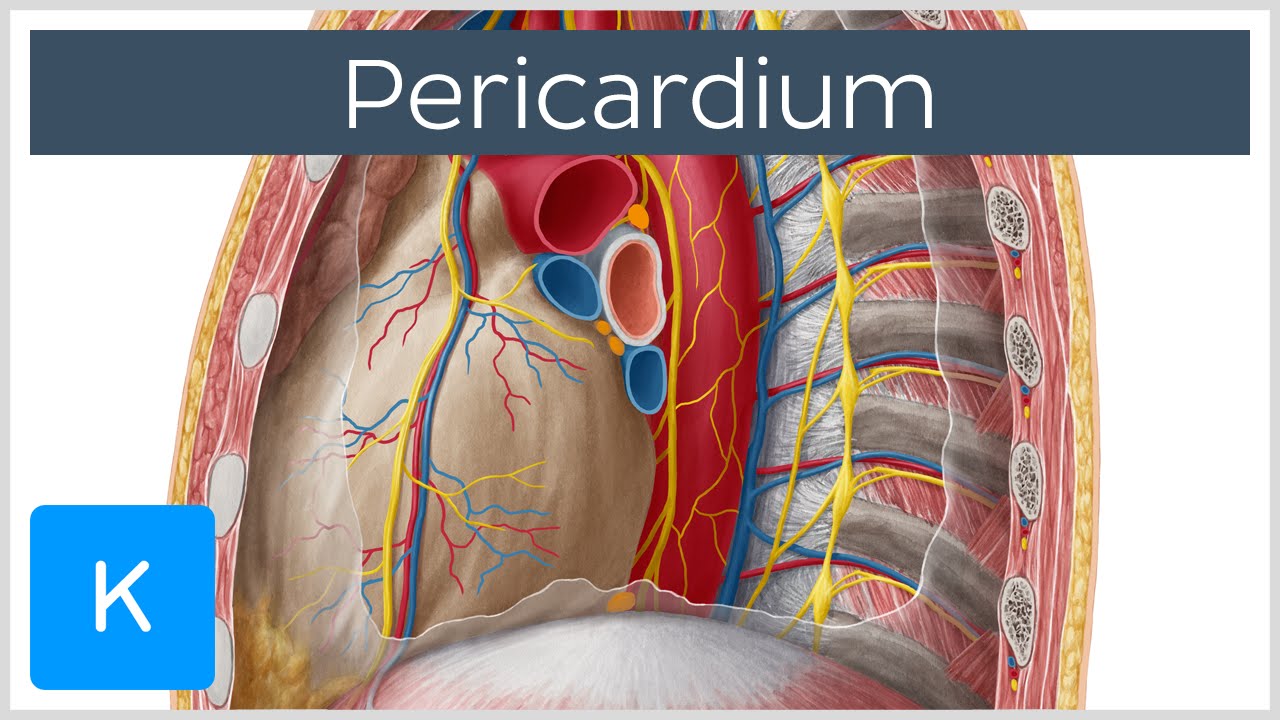This detailed anatomical illustration, most likely hand-drawn using mixed media, depicts a cross-section of the human chest viewed from the side against a white background. At the top of the image, a grayish-purple rectangle with white lettering displays the word "pericardium." The lower right-hand corner features a blue square with a white capital "K." The illustration showcases a complex array of red, blue, and yellow veins and arteries sprawled throughout, alongside a depiction of the heart and possibly lungs, illustrating multiple ventricles and fibrous muscle tissue. Additionally, yellowish areas hint at fat cells, and structures resembling rib bones with visible marrow further enhance the detail. The periphery of the chest section shows layers of bones, muscles, and skin, while orange dots and a white-to-pink gradient diaphragm add further anatomical intricacies.